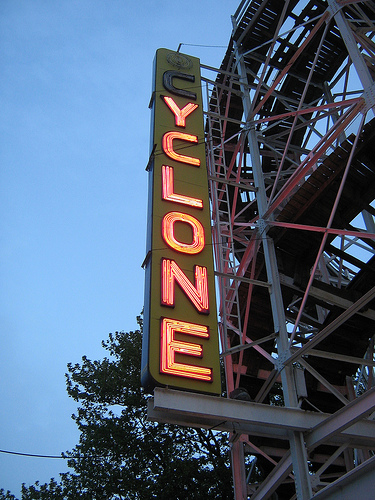This outdoor image captures a neon sign mounted on the metal structure of a roller coaster, likely at an amusement park. The roller coaster's framework is primarily gray with red crossbars, and partial sections of the winding track are visible. The sign, which evokes the retro style of vintage diner signage, has a green background and spells out "CYCLONE" in vertical, red-orange neon letters. Notably, the "C" at the top is unlit. Behind the coaster, there are trees silhouetted against the blue evening sky, hinting at the onset of nightfall. A tall, thin metal ladder is affixed vertically to the right of the neon sign. The overall scene is viewed from a low angle, adding to the towering impression of the ride.